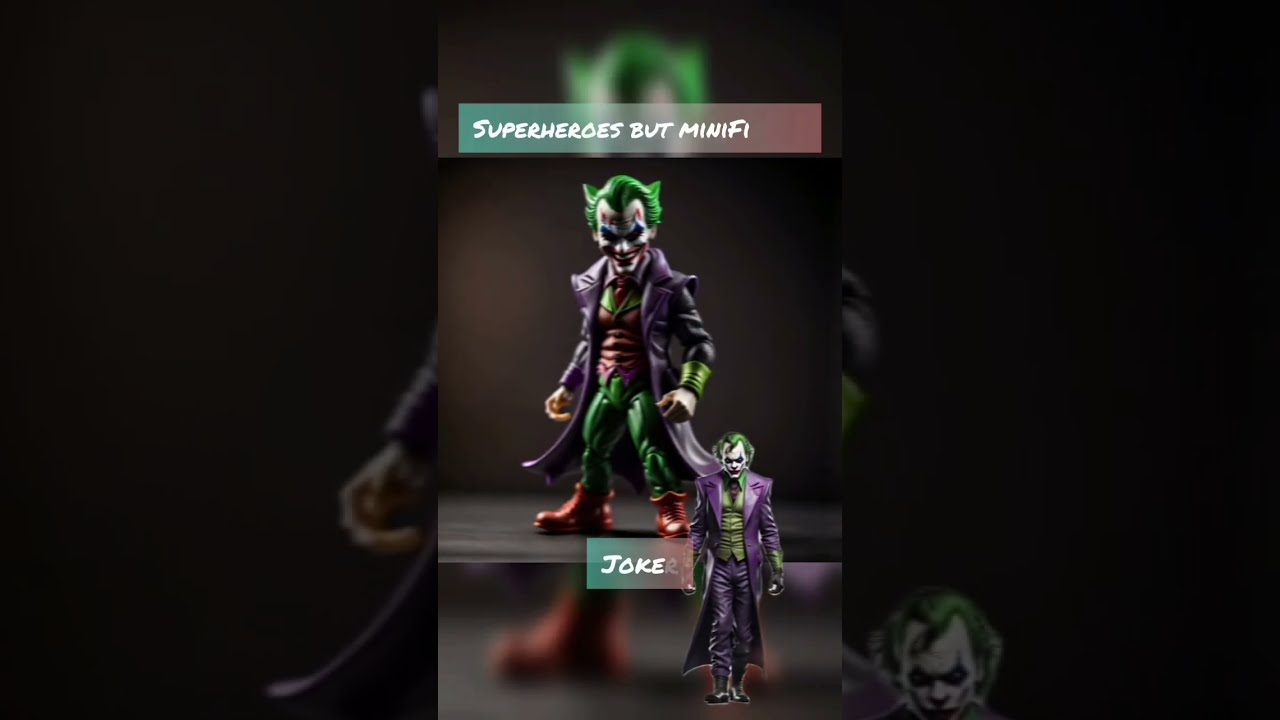The image showcases the Joker from Batman, depicted in two forms. At the top, in an aspect ratio similar to an iPhone screen, text in white reads "Superheroes but Minify." Below this, a large plastic action figure of the Joker stands on a platform. This figure features Joker's iconic green hair, white face paint with red lips, and a sinister clown mask. He is dressed in a distinctive long purple coat, a dark red and green vest, a shirt with a tie, green pants, and either red shoes or brown boots. Directly beneath this figure, the text reads "Joker." In the bottom right, a smaller, more detailed and realistic image of the Joker is seen. This more familiar representation from the comics shows him walking towards the viewer, wearing a purple jacket, a green vest, and black shoes. The background complements the image with a larger depiction of the Joker, enhancing the menacing vibe of the character.